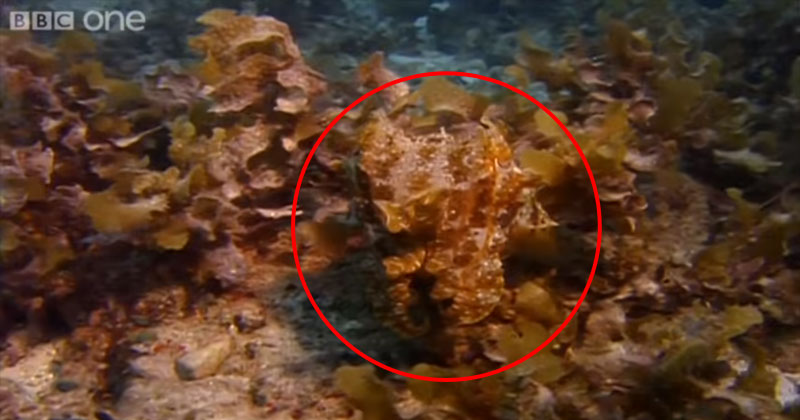The image is a still shot from a BBC One program, most likely a documentary, showcasing an underwater scene. In the upper left-hand corner, there is a white watermark that reads BBC One. The picture captures the ocean floor, where various types of coral and marine plants are visible. The water appears bluish and relatively clear, allowing for a detailed view of the seabed.

At the center of the image, an orangish-red coral is circled with a thin red line, highlighting it as the focal point. This coral is somewhat lumpy and not particularly leafy, distinguishable from the surrounding marine life that includes other corals, green algae, and rocks. The surrounding corals range in color from light brown to brown, and there is a presence of green moss. The scene appears vibrant and slightly blurry, but the highlighted coral in the center stands out against the sandy and rocky backdrop of the ocean floor.